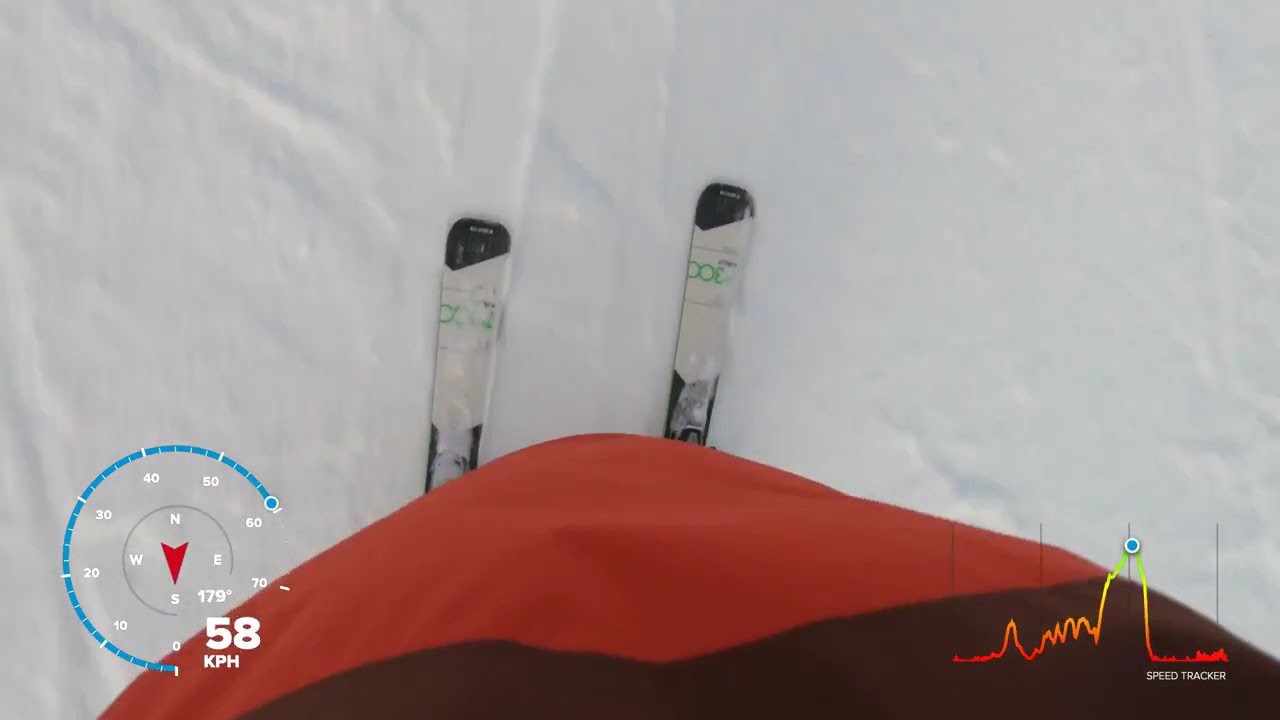The image captures a skier's point of view looking down at their white skis, which feature green markings. The surface beneath the skis is a pristine layer of snow. The skier is dressed in red clothing, prominently visible in the lower third of the photograph. On the bottom left corner of the image, there is an overlay displaying a circular compass, with red pointers and directional markers (N, E, S, W), and a speedometer reading "58 KPH." In the bottom right corner is a speed tracker graph, featuring a curve that changes colors from red to orange, and then to green, representing different speed levels as it oscillates. The overall scene combines detailed instrumentation overlays with the serene, snowy environment of an outdoor ski slope.